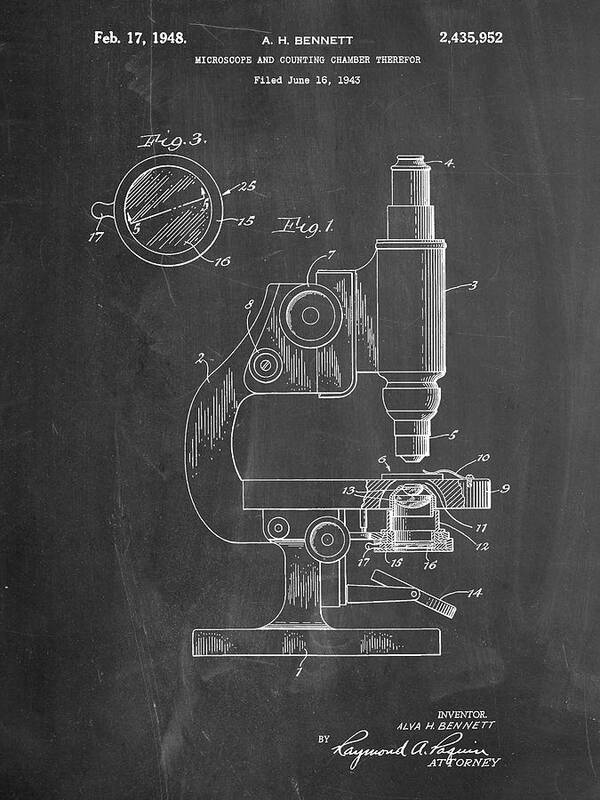This is a detailed black-and-white diagram of a microscope, sketched on a blackboard-like surface with white writing. Dated February 17th, 1948, it displays A.H. Bennett's Microscope and Counting Chamber, noting the filing date as June 16, 1943, and patent number 2,435,952 at the top right. In the top left corner, a figure labeled "Figure 3" shows a circle with a line through it, angled upwards to the right, with arrows pointing to numbers 25, 15, and 16. A horseshoe-shaped line attached to the circle is marked 17. Below this, "Figure 1" identifies the main microscope illustration.

The microscope is in the center, viewed from the side with the eyepiece facing right. The top portion is labeled 4, the cylinder beneath it is 3, and the smaller cylinder below that is 5. A dial to the left of the main cylinder is labeled 7, with a smaller dial labeled 8 below it. The curved portion connecting these parts to the microscope's base is labeled 2. To the right of the microscope, various parts are marked with numbers such as 6, 10, 9, 11, 12, 16, 15, and 17, highlighting parts of the rectangular structure beneath the cylindrical section. A disc labeled 14 extends below this segment, and the base of the microscope is labeled 7.

At the bottom right, the text reads, "Inventor Alva H. Bennett by Raymond A. Pasquale, Attorney," certifying the diagram.